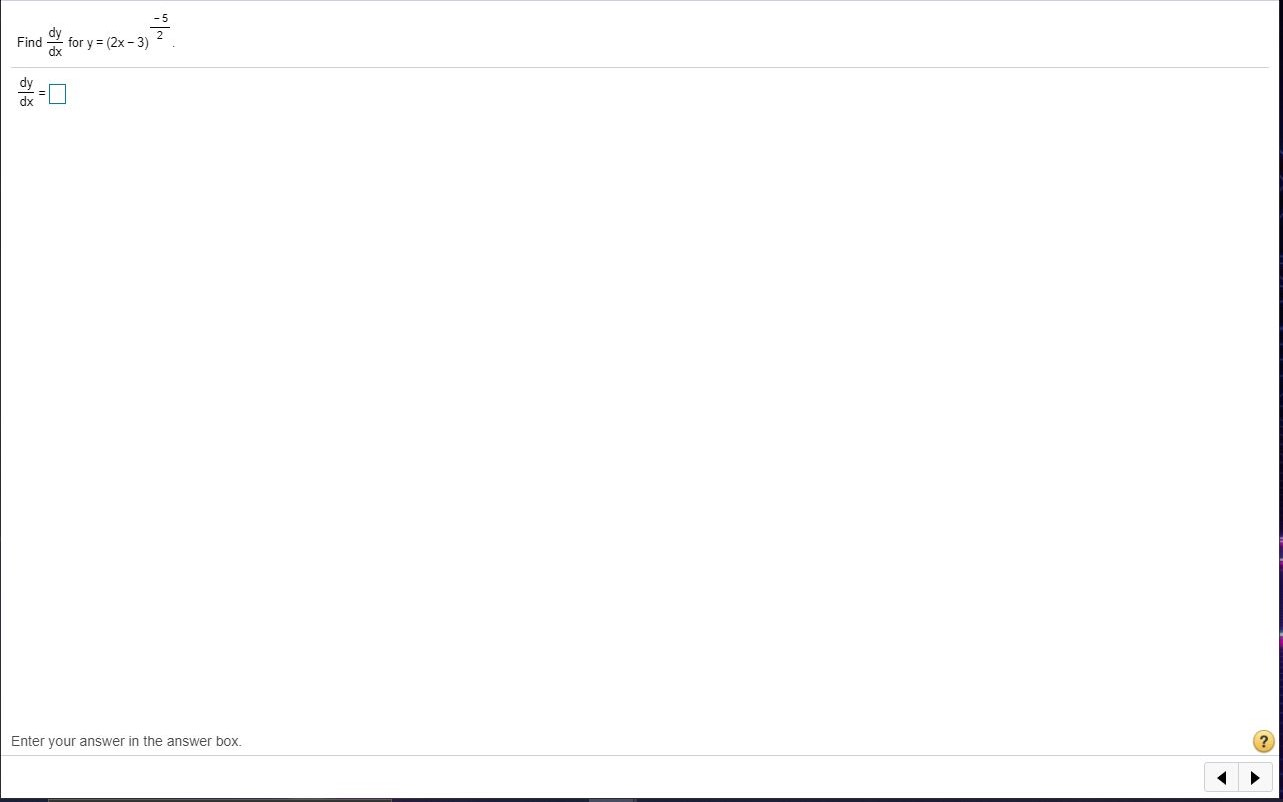The image appears to be a screenshot taken from an educational or mathematical software interface. The primary background of the screenshot is predominantly white, creating a clean and minimalistic appearance.

At the top left corner, an equation is prominently displayed: "Find dy/dx for y = (2x - 3)^(-5/2)." Just below this equation, a light gray horizontal line serves as a visual separator between the question and the answer input section.

Beneath this line, a partially completed equation is visible: "dy/dx = ". Adjacent to this expression, there is a small, empty rectangular box outlined in green, presumably designed as a text field for the user to input their response.

On the lower left side, a clear instruction is written in black text: "Enter your answer in the answer box." The right side of the image features a thick black vertical border, while a similarly thick black horizontal border can be seen along the bottom edge of the screenshot.

In the screenshot's lower right corner, a small yellow circular icon with a black question mark in its center is present, likely indicating helpful tips or assistance. Directly below this icon, there are two light gray, triangle-shaped buttons outlined in darker gray, facing left and right, possibly for navigation purposes.

Additionally, there is a noticeable amount of blank space throughout the image, contributing to the uncluttered feel of the interface. At the very bottom of the screenshot, a text box can also be observed, although the details of its contents are not clearly visible.